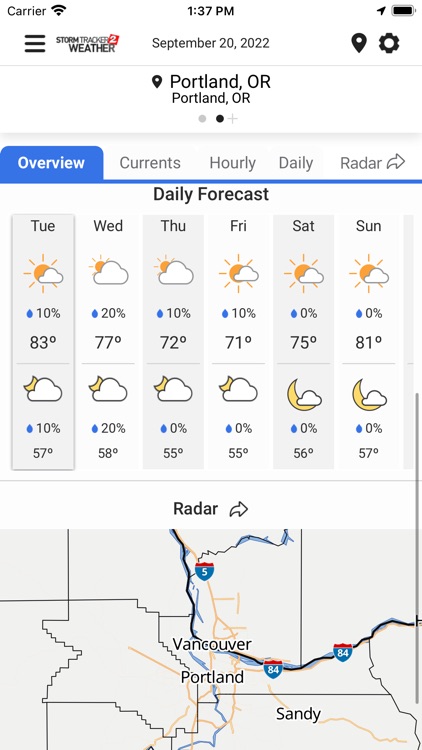Screenshot of a weather forecasting app on a smartphone for Portland, Oregon taken on September 20, 2022, at 1:37 PM. The display shows multiple tabs at the top of the screen: Overview, Currents, Hourly, Daily, and Radar, with the "Overview" tab highlighted in blue. Below these tabs, it shows a section titled "Daily Forecast" with detailed weather predictions for the week:

- **Tuesday**: 10% chance of precipitation, with a high of 83°F. At night, 10% chance of precipitation, with a low of 57°F.
- **Wednesday**: 20% chance of precipitation, with a high of 77°F. At night, 20% chance of precipitation, with a low of 58°F.
- **Thursday**: 10% chance of precipitation, with a high of 72°F. At night, 0% chance of precipitation, with a low of 55°F.
- **Friday**: 10% chance of precipitation, with a high of 71°F. At night, 0% chance of precipitation, with a low of 55°F.

A map is displayed underneath these forecasts showing the geographical layout of Portland, including neighboring Vancouver.